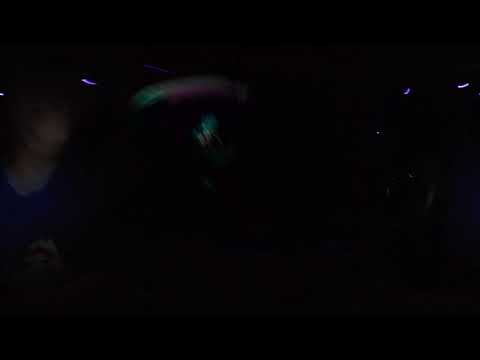This image is predominantly dark with nearly the entire frame appearing pitch black. However, in the top third of the photograph, a series of faint lights can be discerned. On the upper left, there is a violet swipe of light, and nearby towards the center, a larger beige blob becomes more apparent. Further right, an array of colorful fragments, including green and neon pink swipes, are faintly visible. Upon closer inspection, the beige blob in the center reveals the blurred, indistinct face of a person wearing a blue shirt, with outstretched arms suggested by the light on either side. The image appears to have been taken at night, likely outdoors, capturing an almost ghostly impression amidst the darkness.